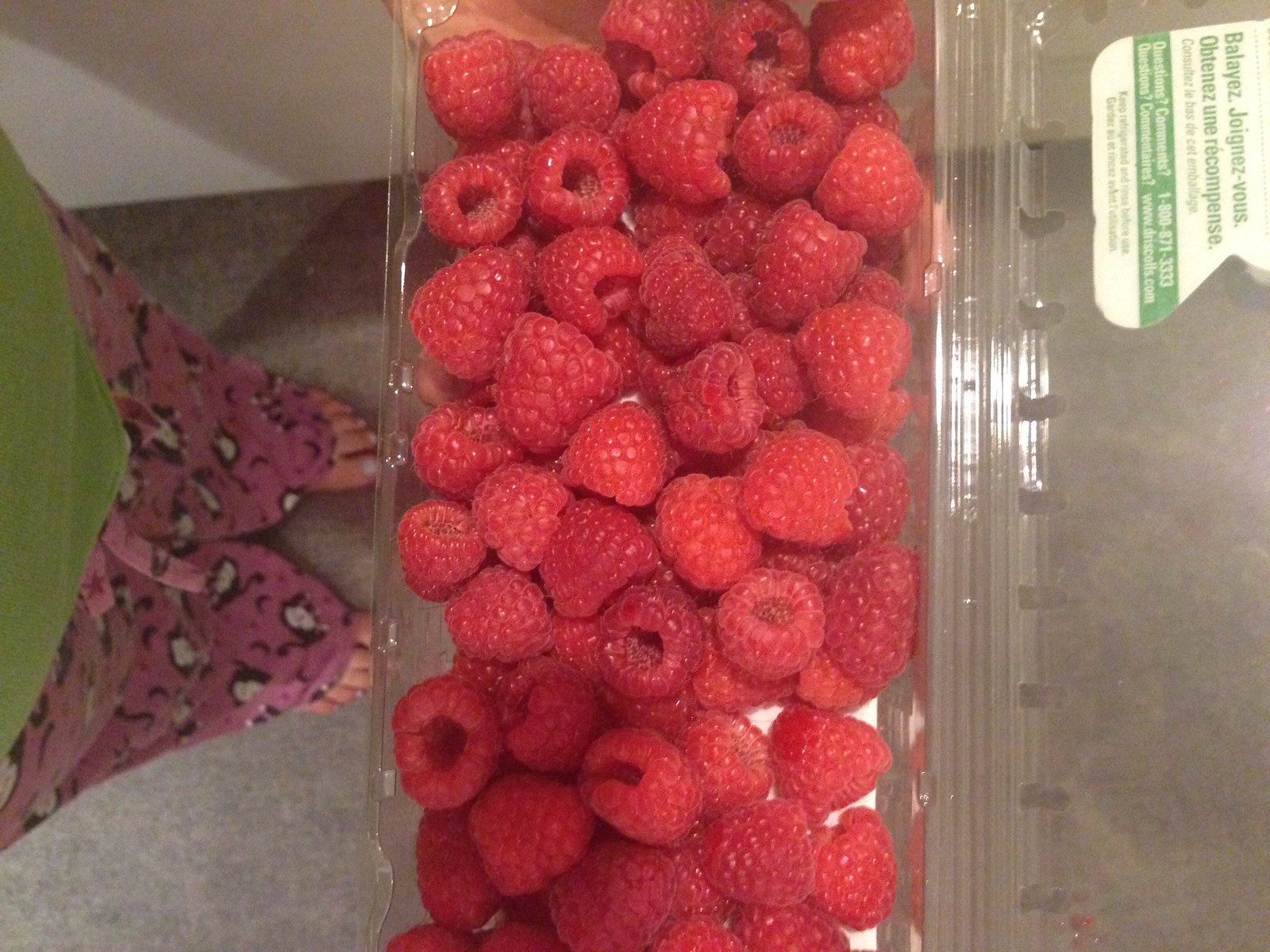In this top-view photograph, a clear, thin plastic container, filled to the brim with bright red raspberries, is being held up by an individual dressed in cozy sleepwear. The container's flimsy lid is opened, revealing the abundance of fresh raspberries inside. The person holding the container is dressed in a green top and pink pajama pants adorned with brown animal prints, which appear to be cats. Beneath their bare feet, a tan carpet extends across the floor. The background features white walls, adding a clean contrast to the image. The hand holding the raspberries and the person’s legs are in full view, capturing a casual, intimate moment centered around the fresh fruit. Subtle details of French writing on the container hint at its contents' origins.